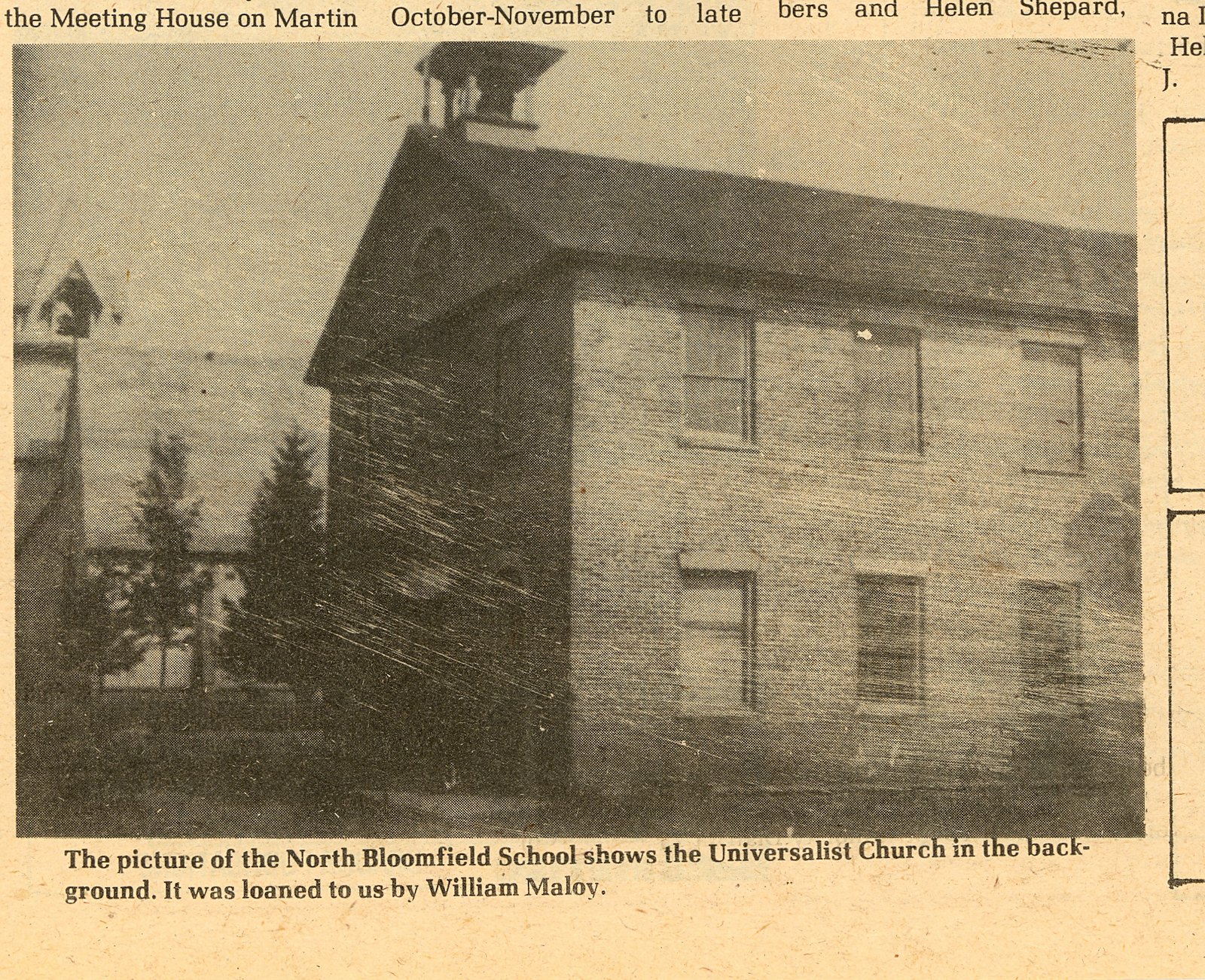This aged sepia-toned newspaper clipping shows a black-and-white photograph of a historic brick building, possibly a church, with a small belfry on the left side and a peaked, sloping roof. The rectangular structure has six visible windows, three on the top and three on the bottom. Evergreen trees are positioned between this building and another structure in the background, where you can also see the church steeple. At the top of the image, in black lettering on the sepia background, it reads: "The Meeting House on Martin, October to November, too late, Burrs and Helen Shepard." The bottom of the image further identifies the scene: "The picture of the North Bloomfield School shows the Universalist Church in the background. It was loaned to us by William Malloy."